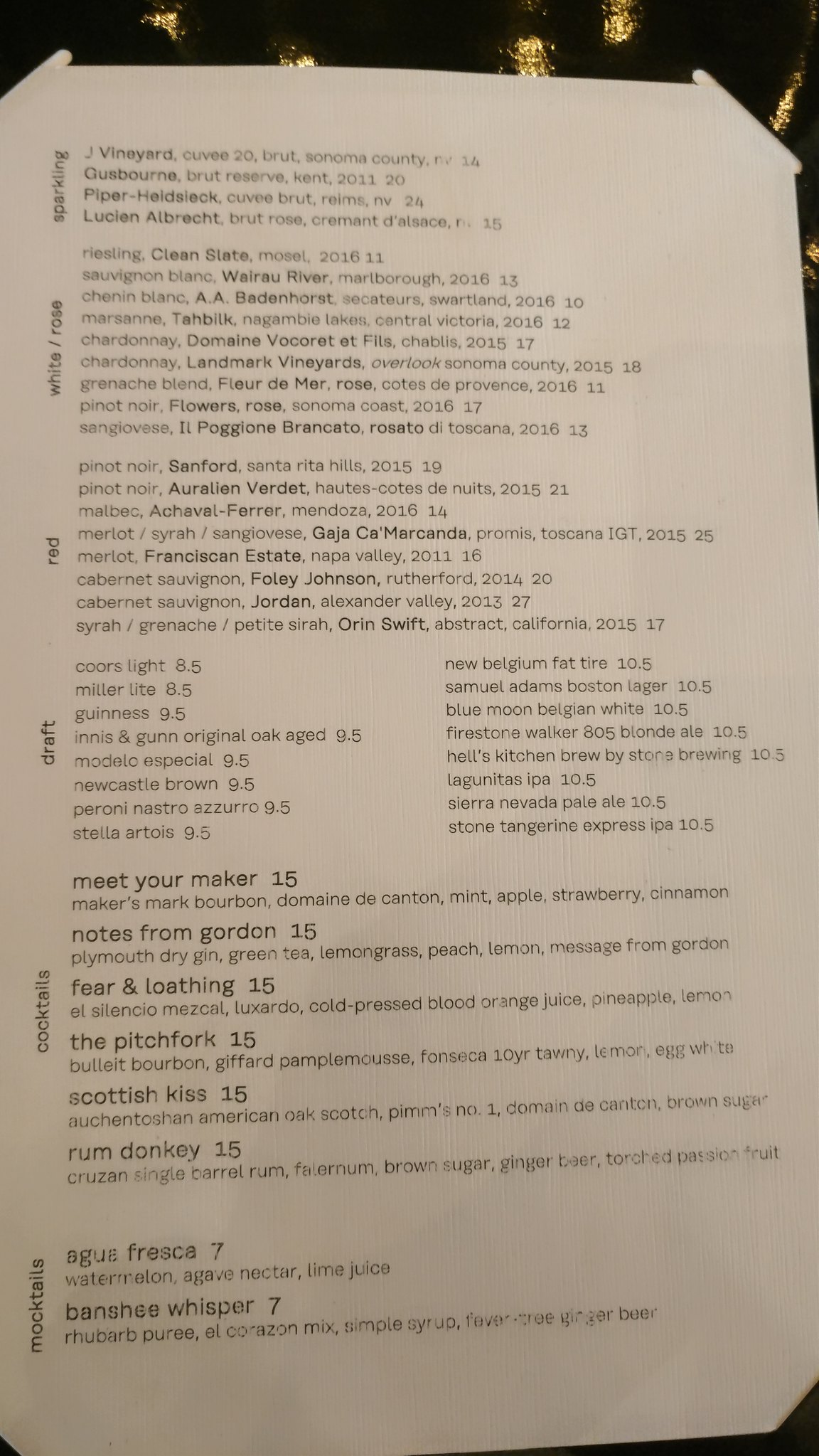This image features a close-up of a piece of paper, prominently positioned as the main subject. The paper appears to be a menu, surrounded by black spots that frame the corners of the photograph. The text on the menu is organized in a somewhat challenging-to-read format due to occasional blurriness. 

A vertical sidebar categorizes the beverages under headings: "Sparkling," "White," "Rosé," "Red," "Draft," and "Cocktails." Adjacent to these categories, the menu lists individual items in horizontal rows. 

In the "Sparkling" section, several beverages are named, including "Vineyard," "Gooseburn," "Piper Hellstick," and "Lucian Albrecht," each followed by an illegible description and a number that presumably represents the price. The "White" and "Rosé" sections contain listings that are mostly unreadable due to the blurriness of the text, with each item similarly followed by a number.

Notably, the "Draft" category differs from the rest by featuring two rows of drinks, implying a more extensive selection. The "Cocktails" section is presented twice, suggesting a possible repetition or sub-category differentiation within this group.

Overall, the menu's presentation is slightly obscured, but the general layout and structure can be discerned from the visible portions.